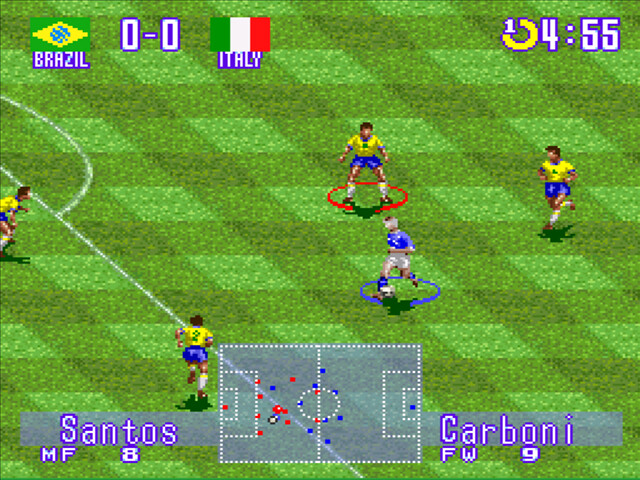This screenshot from an old video game captures a classic soccer match between teams representing Brazil and Italy. The scene, with distinctly pixelated graphics reminiscent of early 80s or 90s video games, features a green football field as the background. The Brazilian team is in yellow shirts and blue shorts, while the Italian team is in blue shirts and white shorts. Four Brazilian players are visible, alongside one Italian player holding the ball. Notably, one player has a red circle around their legs, and another has a blue circle, indicating their active status.

In the top left corner, the flags of Brazil and Italy are displayed with a tied score of 0-0. The top right corner shows a timer at 4:55, alongside a small circle with the number 1. At the bottom of the screen, there's a mini-map of the playing field with blue and red dots marking the positions of team members. Names and roles of players such as "Santos MF8" and "Carboni FW9" are shown within a gray box extending from the map. The screenshot perfectly captures the nostalgic essence of retro gaming with its simple yet detailed depiction of a soccer match.